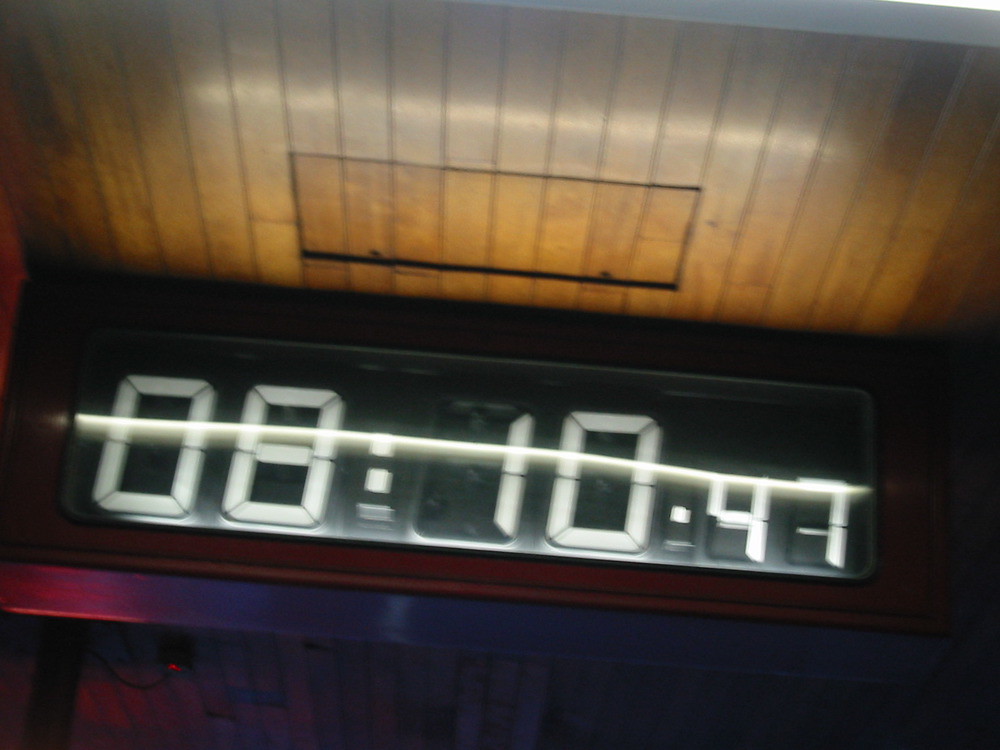This color photograph is a detailed close-up of an old-fashioned digital clock display set against a backdrop of dark wooden paneling. The digital readout, in white on a black screen, shows the time as 08:10:47, with a subtle crack running horizontally through the digits. The display is embedded in a rectangular wooden casing that has a dark, almost black-blue hue towards the right and bottom edges. A small piece of reddish light illuminates the left-hand side of the display. Surrounding the clock are brown wooden planks, with a grey edge visible at the very top, which might suggest a ceiling. The photograph also captures a small black rectangular cutout at the center of the wood panels. An electrical cord extends from a post near the display, plugged into an outlet that emits a red light, adding further intrigue to the scene. The underlighting casts a pinkish tint on some of the wood panels, enhancing the depth and texture of the composition.